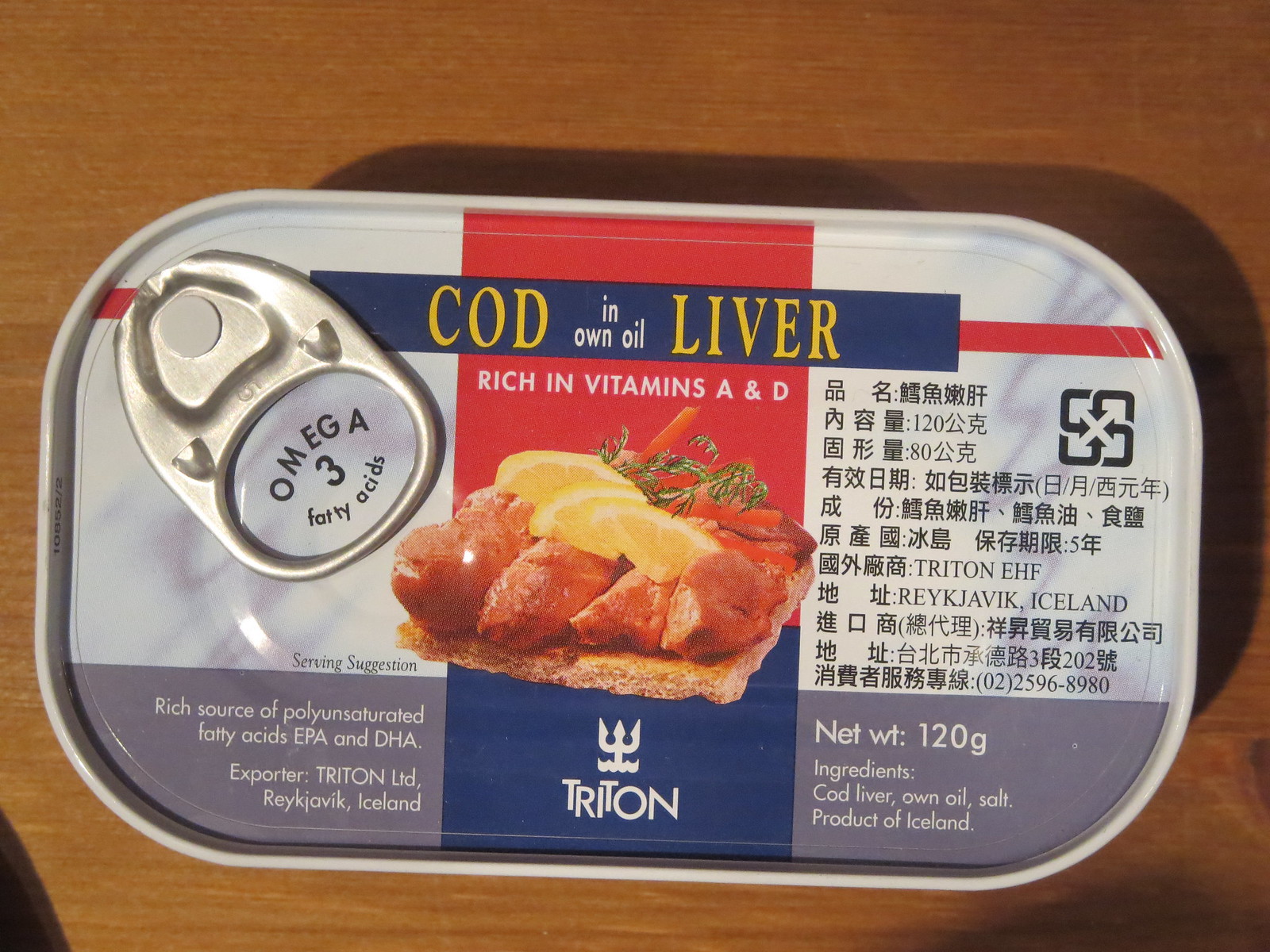The image showcases a pop-top can of cod liver in its own oil, placed on a tan-brown wooden table with visible grain patterns. The rectangular can, with curved sides, features a white label with various colored sections. Prominently, there's a silver pull-tab on the upper left corner. 

Centered on the label is a large red rectangle with the text "cod liver" in yellow. Above this, in a blue rectangle, "cod" and "liver" are again written in yellow, while "in own oil" appears in smaller white font. Just below, the phrase "rich in vitamins A and D" is printed in white within the red section. Additionally, a graphic of cod liver on melba toast garnished with lemon slices, carrots, and parsley emphasizes serving suggestions and the nutritional value, highlighting the presence of polyunsaturated fatty acids, EPA, and DHA.

On the right side, where the label is predominantly white, a circle indicates omega-3 fatty acids. The bottom of the can transitions to a blue section featuring the word "Triton" accompanied by a white fishing spear icon. Below this, export details state "Triton Limited, Reykjavik, Iceland." The net weight is mentioned as 120 grams with ingredients listed: cod liver, own oil, and salt, specified as a product of Iceland. The left side of the can presents additional text in various languages, likely including Chinese, emphasizing the international appeal and distribution of the product.